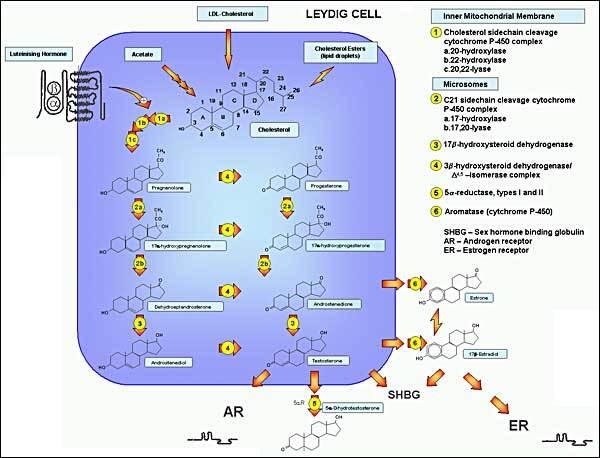The image is a detailed diagram from a textbook or scientific magazine, labeled "Leydig Cell" at the top. Encapsulated in a large blue square with rounded corners, the image contains various molecular structures and honeycomb-like representations, each carefully labeled to illustrate different chemical bonds and components. Numbered red arrows with yellow circles highlight the actions and processes occurring within the diagram. To the right of the blue square, there are annotations discussing the inner mitochondrial membrane, including terms like cholesterol side chain cleavage and cytochrome P450 complex, with sub-components like 20-hydroxylase, 22-hydroxylase, and 20,22-lyase. Below this, additional terms like microsomes and C21 side chain cleavage are mentioned along with different enzymes including 17-hydroxylase and 17,20-lyase. The background of the image is white, while the blue square contains compounds and numerous text boxes explaining the mechanical processes. A legend at the bottom helps to distinguish the various parts of the diagram. The overall design is neat, outlined by a thin black square to give a clean finish, and the quality of the illustration is fairly good.